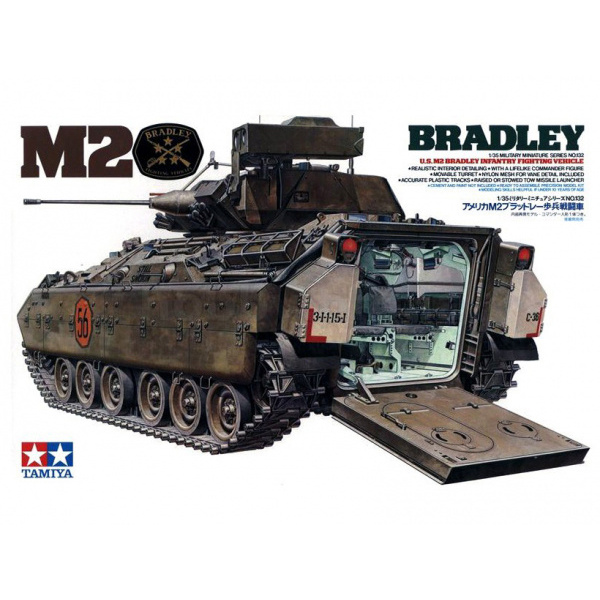This is a colored illustration of the box art for a Tamiya model kit featuring a detailed depiction of an M2 Bradley Infantry Fighting Vehicle, an advanced version of the Bradley personnel carrier. The image showcases the rear view of the vehicle with its back hatch open, revealing a teal blue interior devoid of any crew. The exterior of the tank is painted brown with additional equipment visible on both the turret and the sides of the vehicle. Notably, there is a red circle with black numbers "56" prominently displayed on the side. The turret is oriented towards the front. In the upper right corner, "BRADLEY" is written in black. The Tamiya logo, characterized by a red and blue square with white stars, is located in the bottom left corner. Above the logo, "TAMIYA" is written in capitalized blue letters. Some Japanese text is also present, indicating the likely dual-language nature of the packaging. Additionally, the tank's side features various inscriptions, including "3-1-1-1-5-1" on a gray fuel tank, alongside red L-shaped markings.